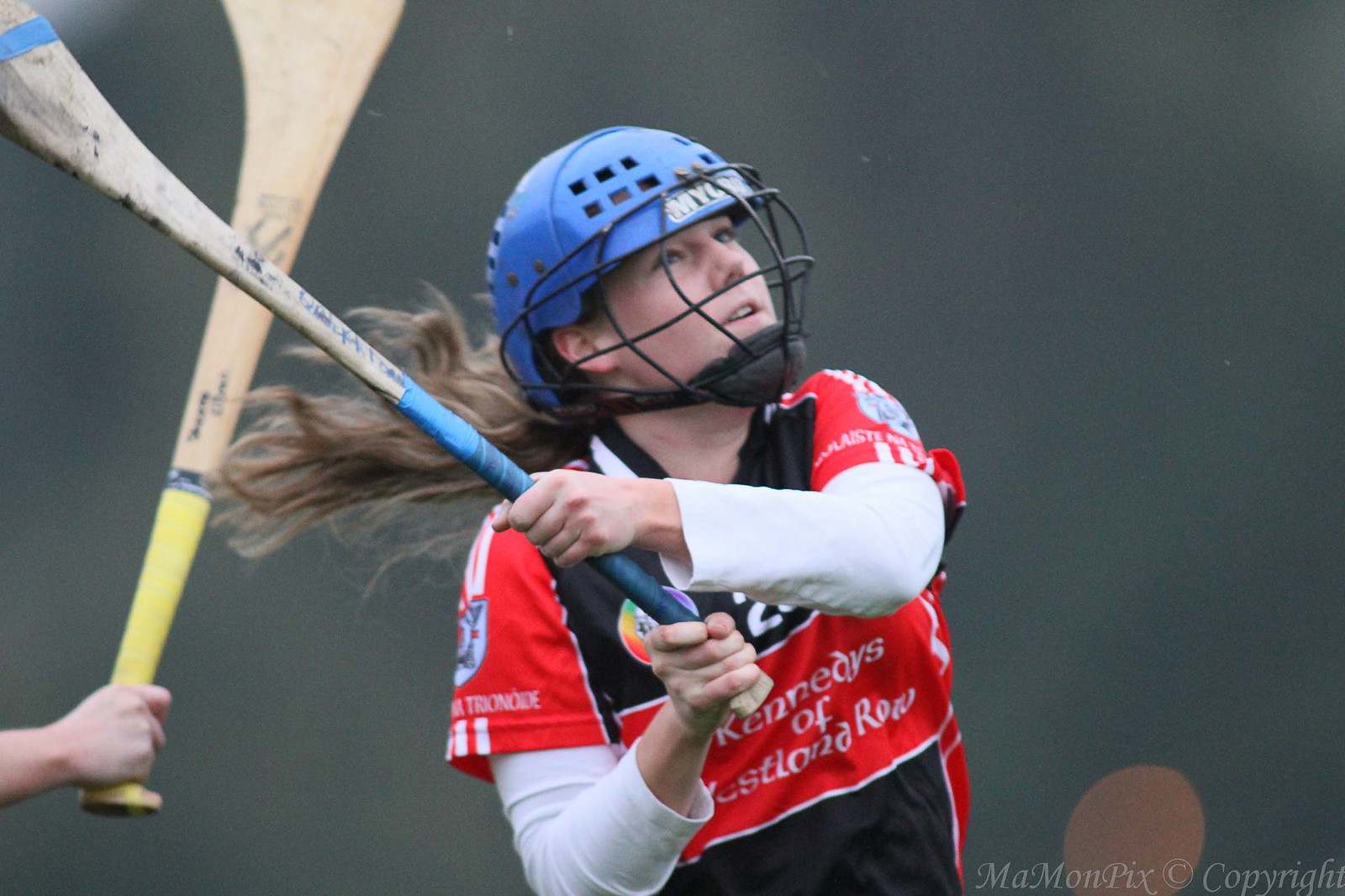The image captures a dynamic moment centered on a female athlete, likely engaged in a competitive sport such as field hockey. The background is a deep gray, which contrasts with the vivid attire of the athlete. She stands prominently in the middle of the frame, shown from the waist up in an action pose. The athlete is donning a blue helmet equipped with a black caged face guard and a chin strap for protection. Her outfit consists of a white long-sleeve shirt layered beneath a short-sleeve red and black jersey, which has white text that appears to read "Kennedy's of Westland Grove," though some of the wording is obfuscated by the wrinkles in the fabric. 

In her hands, she grasps a field hockey stick with blue grips and a flattened, medium-brown wooden head. Another similar stick, this one featuring a yellow grip, intrudes into the frame from the left side, held by an unseen person. The athlete's hair is tied back in a ponytail, and at the bottom right corner of the image, a small watermark reads "MAMONPIX Copyright."